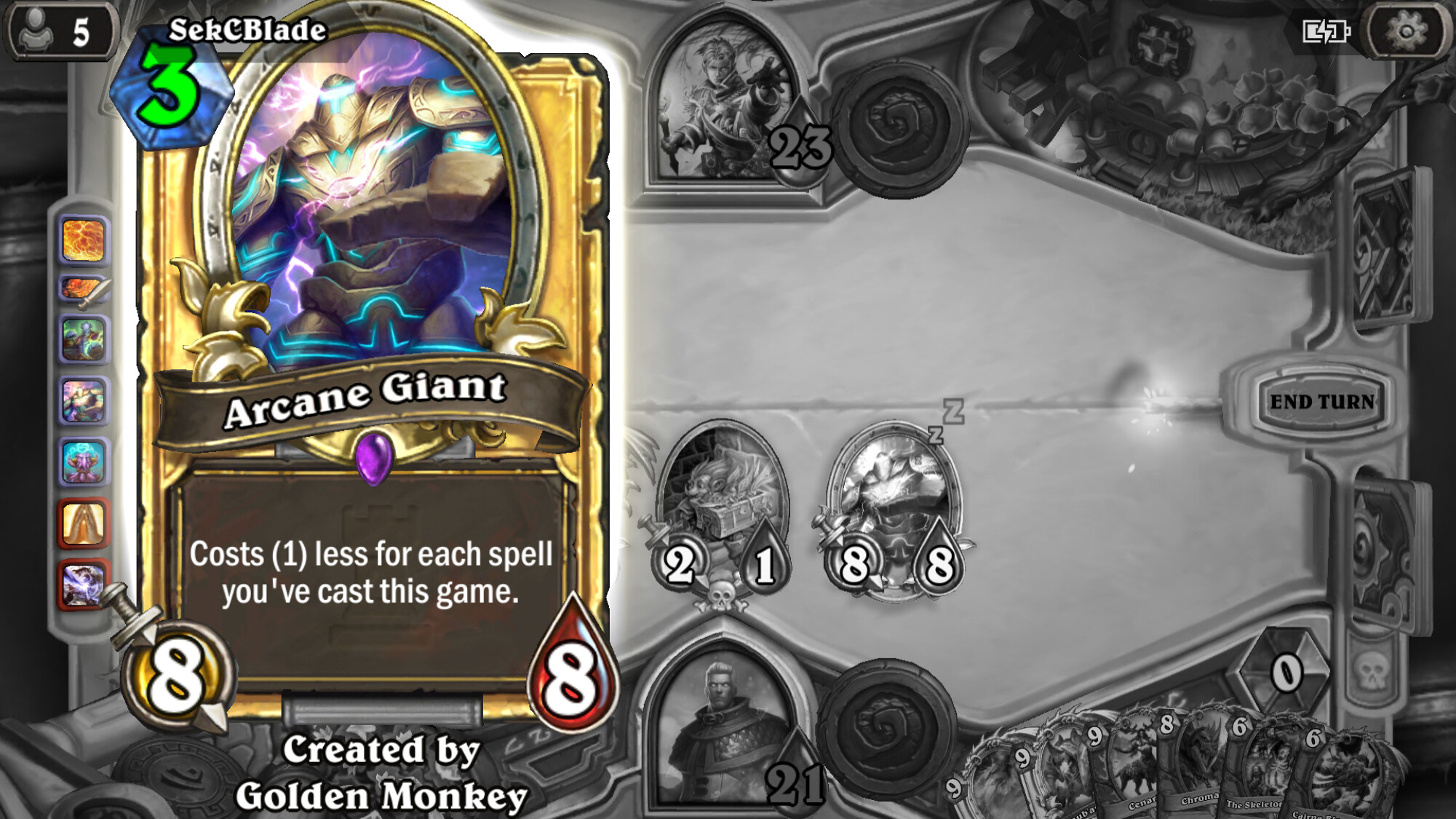This detailed screenshot from a video game features an interface with various elements. In the upper left corner, there is a gray box displaying the silhouette of a person with a white number "5" next to it. To the right of this box, the text "S.E.K. Seablade" is displayed in white font. The background is predominantly black and white, resembling a game board, with two archway windows on either side. One window shows a character with the number "23" next to it, while the opposite window has another character with the number "21."

To the left side of the image, there is a detailed card titled "Arcane Giant." The card's frame is gold with an oval illustration depicting a large, metallic-looking giant adorned with purple and green lightning streaks and green lines on its body. The upper left corner of the card features a green diamond shape with the number "3" inside it. The bottom left corner of the card has an eight in white on a sword-emblazoned sphere, and the bottom right corner shows a white number "8" on a red teardrop shape. Below the image of the giant, on a brown banner, it says "Arcane Giant" in white letters. Beneath this, on a brown box, it explains, "Cost one less for each spell you’ve cast this game." Additionally, the text "Created by Golden Monkey" is noted below the card description. The right side of the image also indicates a battery level icon showing approximately 80% charged. The score is displayed as "8" to "8," with the second "8" inside a red teardrop shape.